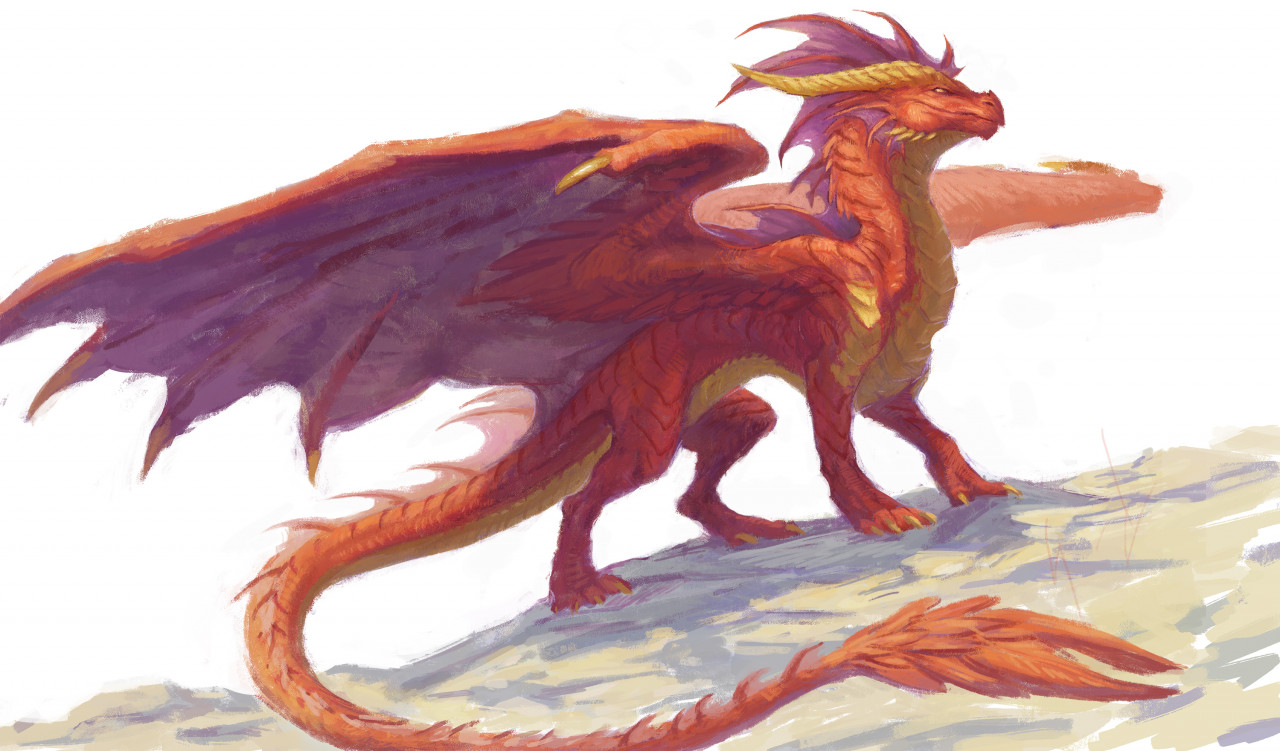The painting depicts a formidable dragon reminiscent of those found in fantasy comics, endowed with the ability to breathe smoke. The dragon's lengthy tail culminates in a bushy, vibrant orange tip. Its body showcases an intricate color palette—bearing a bright yellow underside and distinct orange head. The creature's four limbs, arranged in a stance similar to that of a quadrupedal animal, exhibit sharp yellow claws tipped menacingly. 

Large, widespread wings extend from its back, displaying a striking purple hue on their undersides and featuring unique claws at their tips. The dragon’s head is adorned with a striking mixture of colors: a band of yellow just below the head transitions into a vivid mohawk of purple and orange. The creature's gaze is unnervingly intense, adding to its ominous aura.

The dragon stands on a piece of land that slopes gently, its rocky and earthy brown terrain providing a stark contrast to the vibrant hues of the dragon. The overall scene embodies a blend of vivid colors and intricate details, evoking a sense of otherworldly majesty and latent danger.